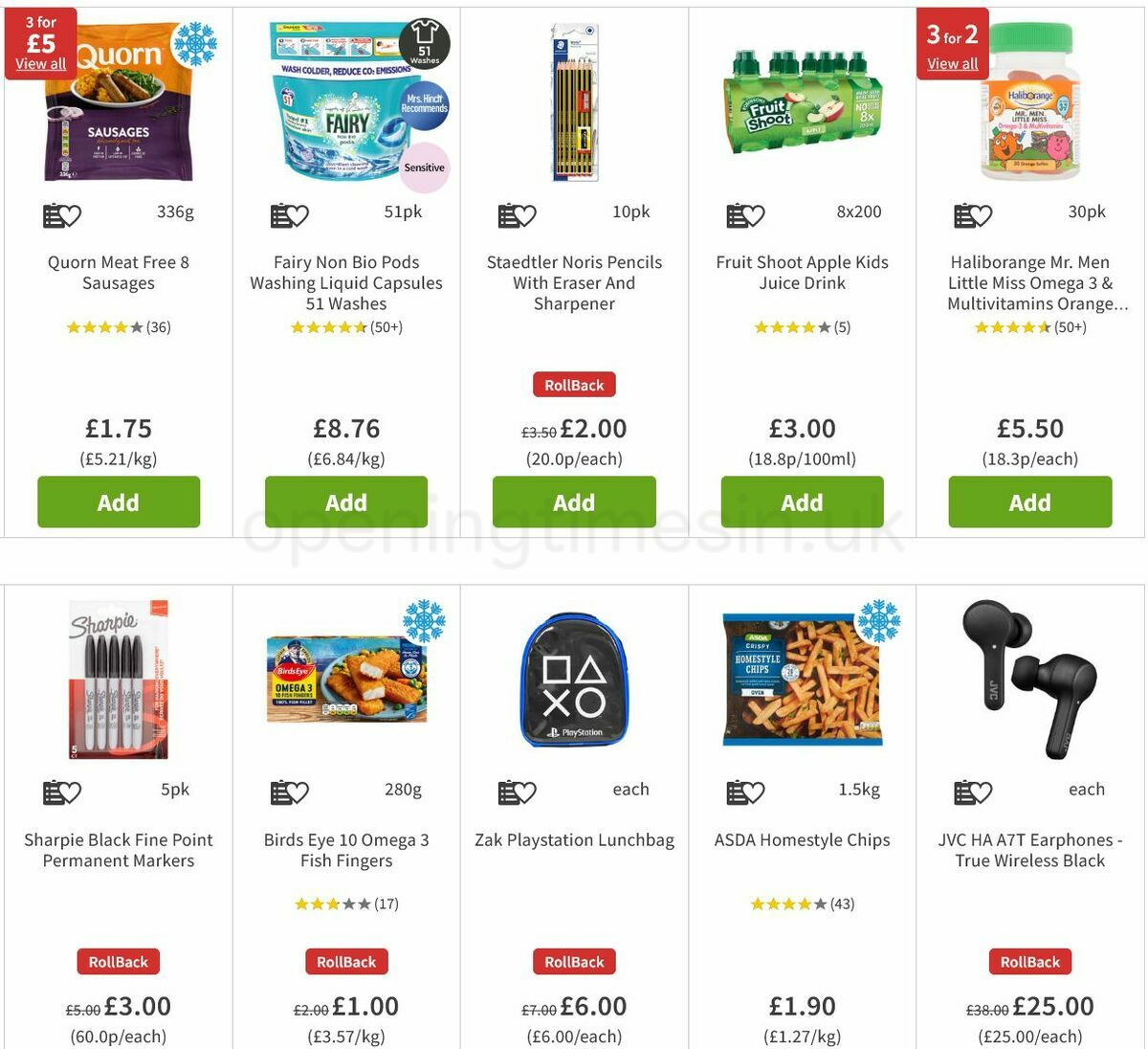This image features a variety of grocery items neatly organized in two rows, with five items on the top row and five on the bottom. The assortment includes a mix of food products, household essentials, and miscellaneous items typically found in a grocery store.

- **Top Row**:
  1. **Quorn Meat-Free Sausages**: Plant-based sausages, ideal for vegetarian or vegan meals.
  2. **Fairy Non-Bio Pods**: Laundry washing liquid capsules, gentle on skin.
  3. **Staedtler Norris Pencils**: High-quality pencils for writing or drawing.
  4. **Fruit Shoot Apple Kiss Juice Drink**: A refreshing apple-flavored beverage.
  5. **Haliborange Mr. Men Little Miss Omega-3 Multivitamins**: Nutritional supplements for children.

- **Bottom Row**:
  1. **Sharpie Black Fine Point Permanent Markers**: Permanent markers perfect for labeling and art projects.
  2. **Bird's Eye Omega-3 Fish Fingers**: Nutritious fish fingers enriched with Omega-3.
  3. **ZAC PlayStation Lunch Bag**: A themed lunch bag featuring PlayStation graphics.
  4. **ASDA Home Style Chips**: Crispy and tasty home-style chips.
  5. **JVC HA-A70T True Wireless Earphones**: Black, wireless earphones for a seamless audio experience.

Each item is labeled with its respective price, which ranges from £1.00 to £50.00, indicated in either pounds or euros. Several items feature red "rollback" stickers, suggesting a discount, and all items have star ratings and heart symbols for adding to favorites. Notably, the Omega-3 multivitamins are marked with a "3 for 2" offer, inviting shoppers to buy two and get one free.